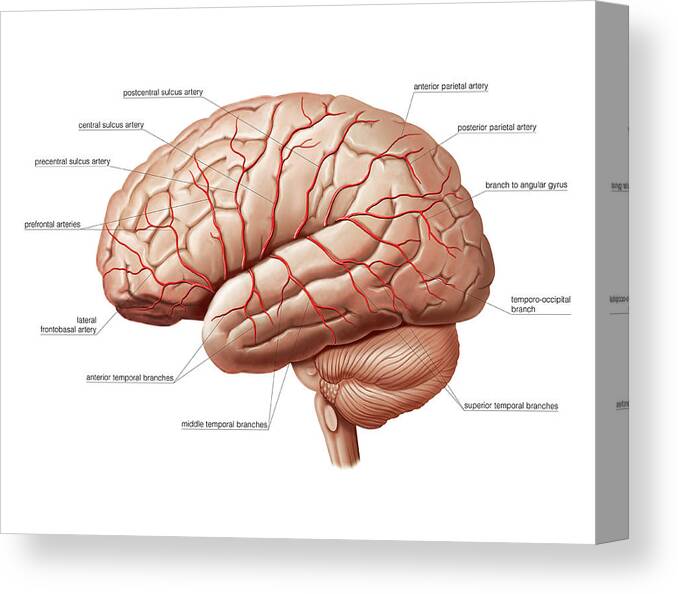This image is a detailed illustration and diagram of a human brain, rendered from a side view and superimposed onto a three-dimensional canvas-like background, marked by a distinctive gray strip running along the right side. The brain itself is predominantly pinkish or light fleshy in color and meticulously labeled with various arteries. These arteries, illustrated in medium red, include the anterior parietal artery, posterior parietal artery, branch to angular gyrus, temporal occipital branch, superior temporal branches, middle temporal branches, anterior temporal branches, lateral frontobasal artery, prefrontal arteries, precentral sulcus artery, central sulcus artery, and postcentral sulcus artery. Each label is connected to its respective part of the brain via fine lines, making the intricate vascular structure of the brain visible against a plain white background. The illustration also includes a detailed depiction of the brainstem, further enhancing the anatomical accuracy and educational value of the image.